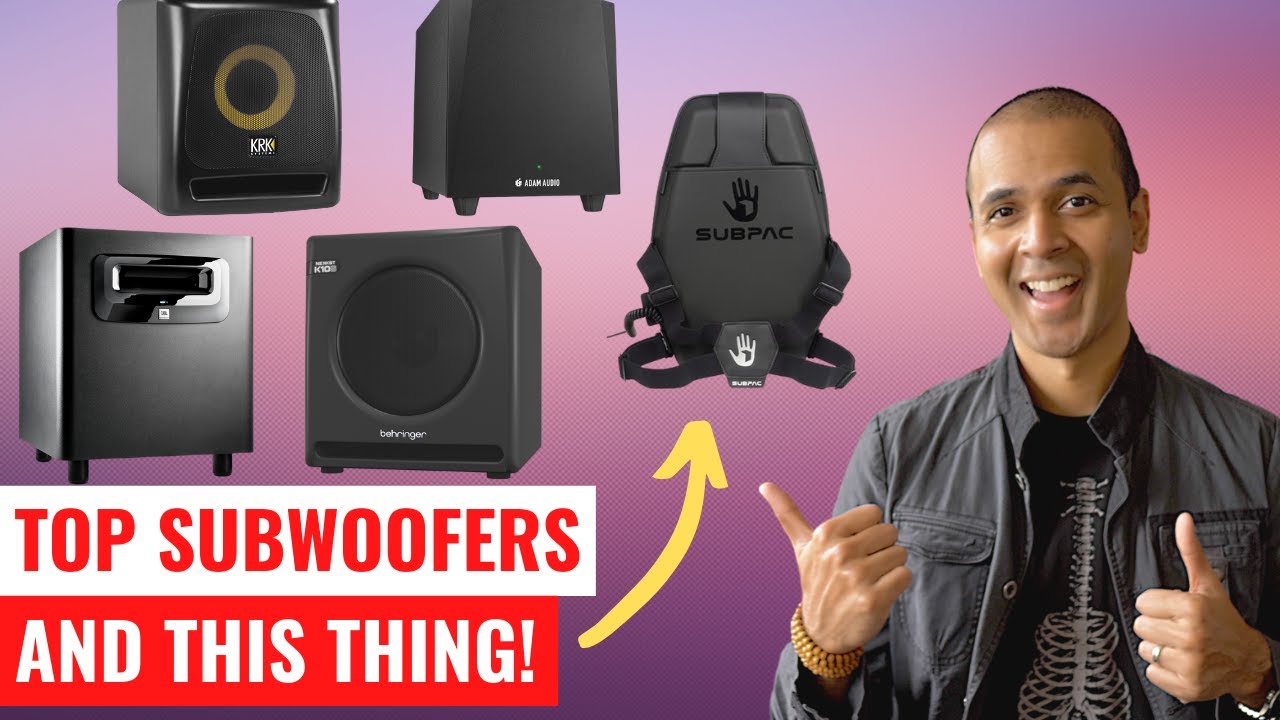The advertisement features a cheerful man with a light-dark complexion, sporting a closely shaved hairstyle. He is dressed in a black button-up shirt over a graphic T-shirt that resembles a guitar made of skeleton bones, and accessorized with a gold bracelet. He's giving a thumbs-up with both hands, with his right thumb also pointing at various subwoofers displayed around him. The background is a gradient of purple and pink, enhancing the dynamic presentation.

On the top right, four boxy black subwoofers from various companies are prominently displayed. Another device, resembling a backpack and labeled "sub pack," stands out. In the bottom left corner, bold white text on a red background reads, "Top subwoofers and this thing," with a yellow arrow pointing from this caption to the "sub pack," highlighting its unique presence among the subwoofers. The overall scene suggests a vibrant, eye-catching ad, possibly for a YouTube thumbnail or a social media post, aimed at showcasing top subwoofers and the intriguing "sub pack" device.